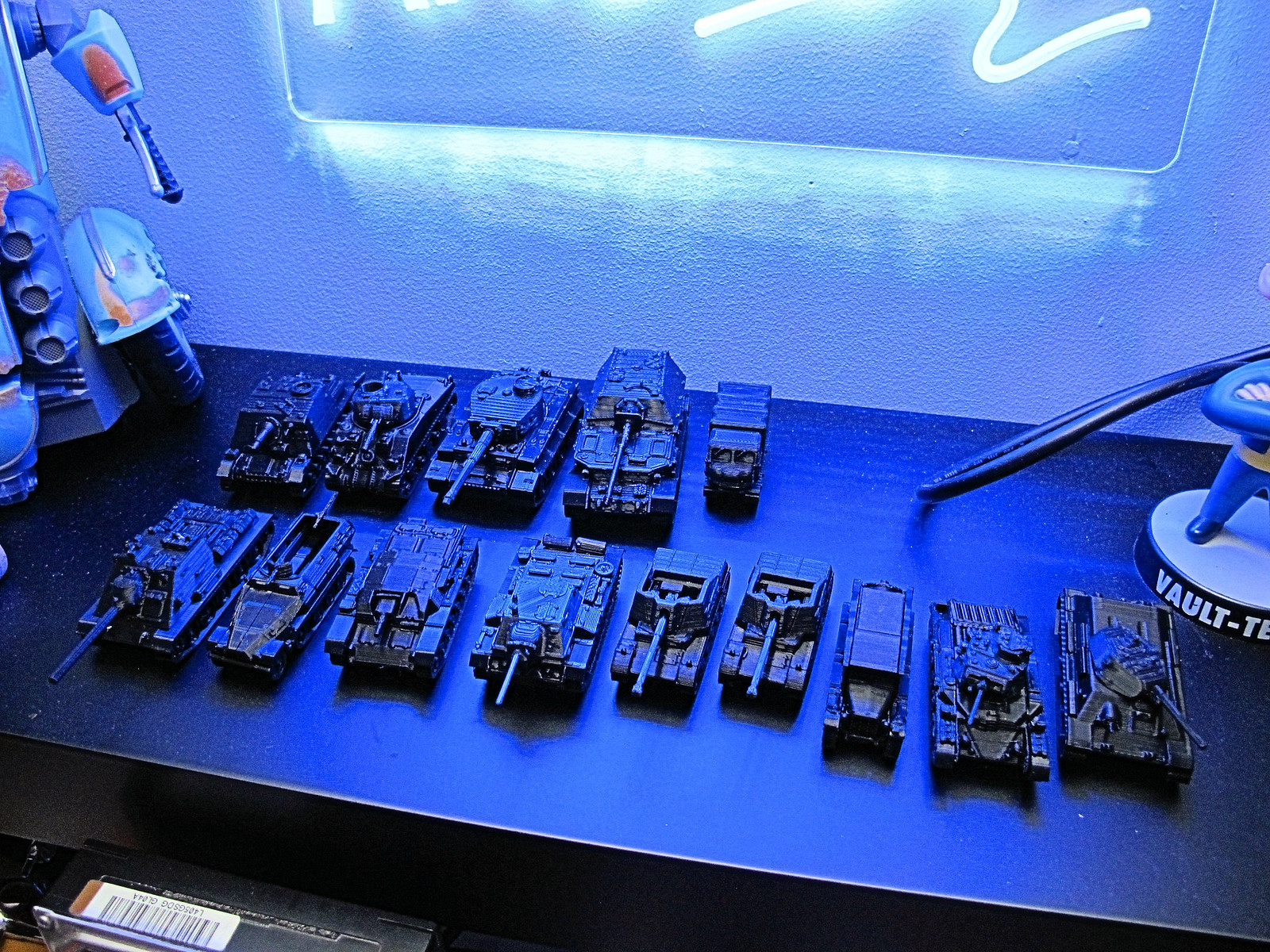The photograph captures a meticulously arranged display of vintage toy army vehicles, including detailed models of tanks, troop carriers, half-tracks, and trucks. The vehicles, all a dark, almost black shade, are presented in two neat rows on a dark blue shelf, resembling a display a child would play with. Each vehicle, from small to quite large, features intricate details such as front rubber wheels, back tracks, and long-range artillery mounted on some tanks. In the back row, four tanks and a truck are lined up, while the front row includes another nine vehicles, predominantly tanks, all parked parallel and facing forward. The background showcases a wall with textured paint, adorned with an illegible neon sign that emits a white, squiggly line of light. Various other collectibles are stacked to the left, and on the right, a pedestal base with a superhero figure stands next to a circular object labeled "vault" and what seems to be a silver machine with knobs. The overall scene is set against a light blue background, enhancing the visibility and historical charm of the miniature army vehicles.